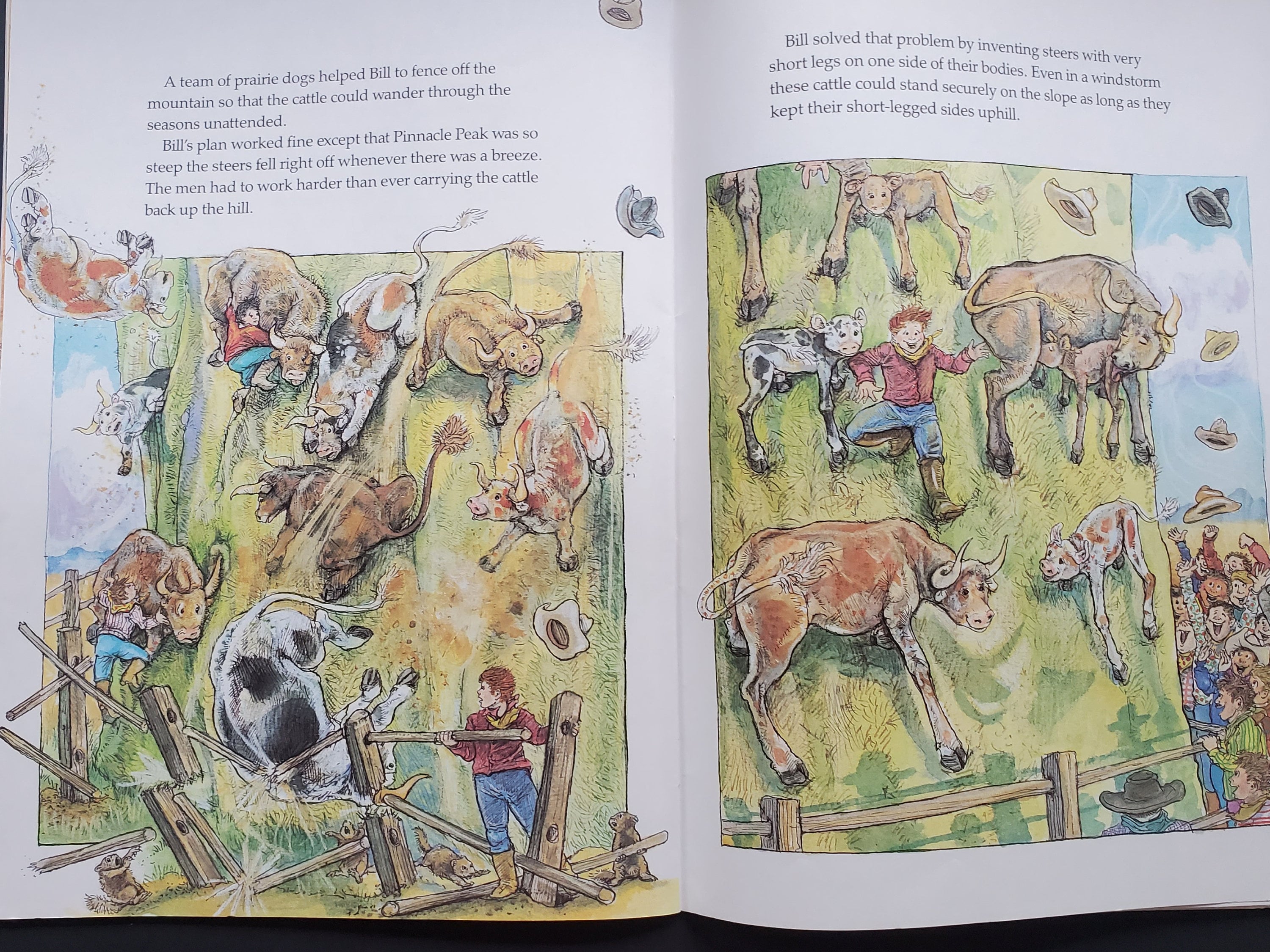The open pages of a children's picture book reveal a lively scene of cows sliding down a steep mountain. On both pages, detailed illustrations capture the chaos: on the left, a couple of men and boys desperately try to fix a broken fence and stop the cows, who are tumbling down the hill. The text explains that prairie dogs initially helped Bill fence off the mountain, but the steep Pinnacle Peak caused the cows to fall whenever there was a breeze. On the right page, more cows are shown stuck half-way down the mountain, while a crowd of people at the bottom cheers and howls, throwing their hats in the air. The narrative humorously notes that Bill eventually solved the problem by inventing cows with short legs on one side, enabling them to stand securely on slopes even in windstorms.